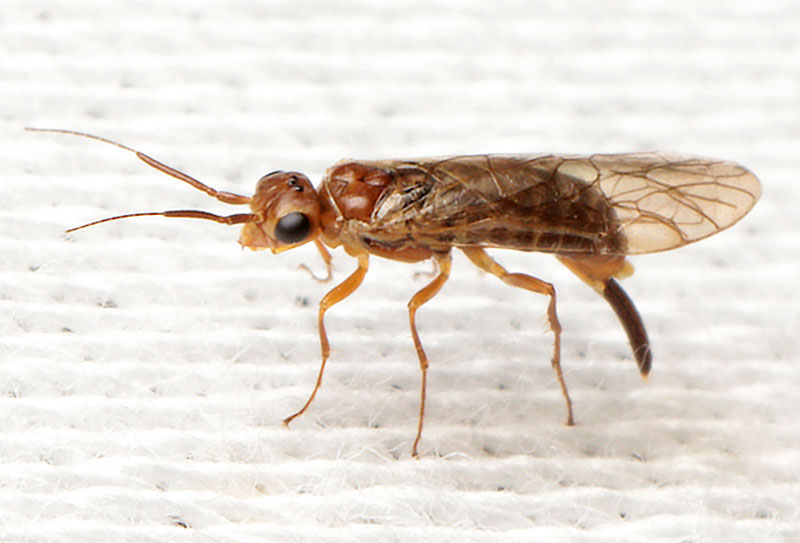This photograph is a detailed close-up of a flying insect, specifically a sawfly, resting on a white ribbed surface, likely a piece of cloth or paper. The sawfly, positioned centrally in the rectangular image, boasts a medium to dark reddish-brown coloration, which deepens towards the rear of its long, segmented body. The insect's six light brown legs, adorned with fine hairs, contrast slightly with its darker body and head. Prominent transparent wings, extending from just behind its head to past its back, display intricate veiny patterns. Notably, the insect's large black eyes, taking up nearly a third of its head, are clearly visible in this up-close left side profile shot. Its long, dark brown antennae curve distinctly from the top of its head, adding to the detailed minimalistic composition of the image.